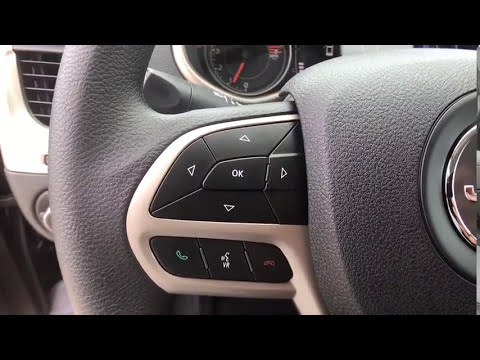The image depicts an extreme close-up of the left side of a black steering wheel within a vehicle, framed in a letterbox format with black bars at the top and bottom. The focus of the shot is on the tactile control buttons embedded in the steering wheel, which are divided into two main groups. The upper group consists of a central "OK" button surrounded by four directional arrows: up, down, left, and right. Below this array, there are three additional buttons: a green phone icon on the left, a red phone icon on the right, and a white symbol in the middle, possibly a speaker. The steering wheel itself has a stucco-like texture. In the background, partially visible through the steering wheel’s openings, are a tachometer from the gauge cluster, a turn signal lever, and an air conditioning vent to the left, along with the gap between the door and the dashboard. The central logo on the steering wheel is cut off and indiscernible due to the close-up nature of the image.